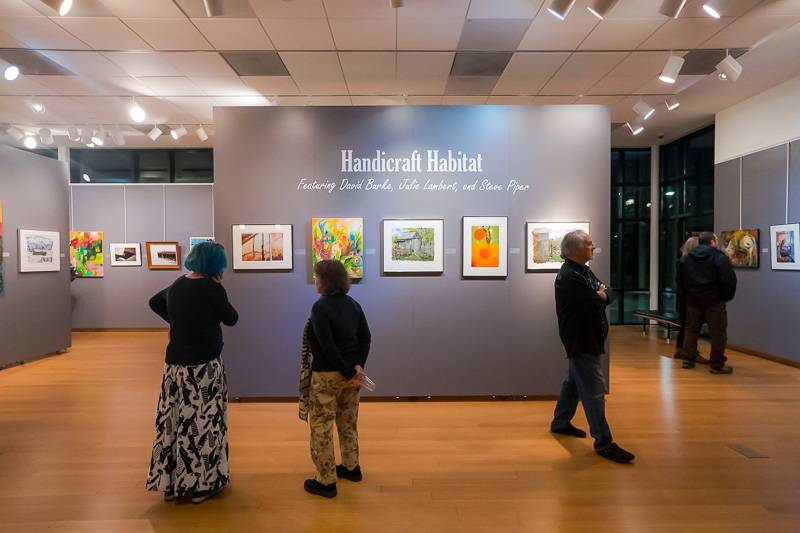This detailed photo captures an art gallery exhibit titled "Handicraft Habitat" featuring artists David Bartle, Jake Landbert, and Steve Piper. At the center of the image, a prominent wall showcases five framed artworks with a background of white and grey letters, announcing the exhibit's title and featured artists' names. The gallery space is well-lit with round, white lights mounted on a white-tiled ceiling, each light focusing on individual art pieces. 

The floor is wooden, creating a warm contrast to the clean, silver-toned background that defines each artwork. On the left side of the image, two women are closely observing a piece; one has striking blue hair, wearing a black shirt and a black and white skirt, while the other wears a black top, white pants, and black shoes, with her hands clasped behind her back. To their right, a gray-haired man stands with his arms folded, appearing deep in thought as he walks by the exhibits.

On the far right, a couple attentively examines another piece of art. The space feels alive with the movement and engagement of these visitors, set against a backdrop of meticulously arranged artworks, each suspended by white strings against the silver canvas-like background. The overall scene conveys a serene yet engaging atmosphere as patrons take in the diverse artistic expressions on display.